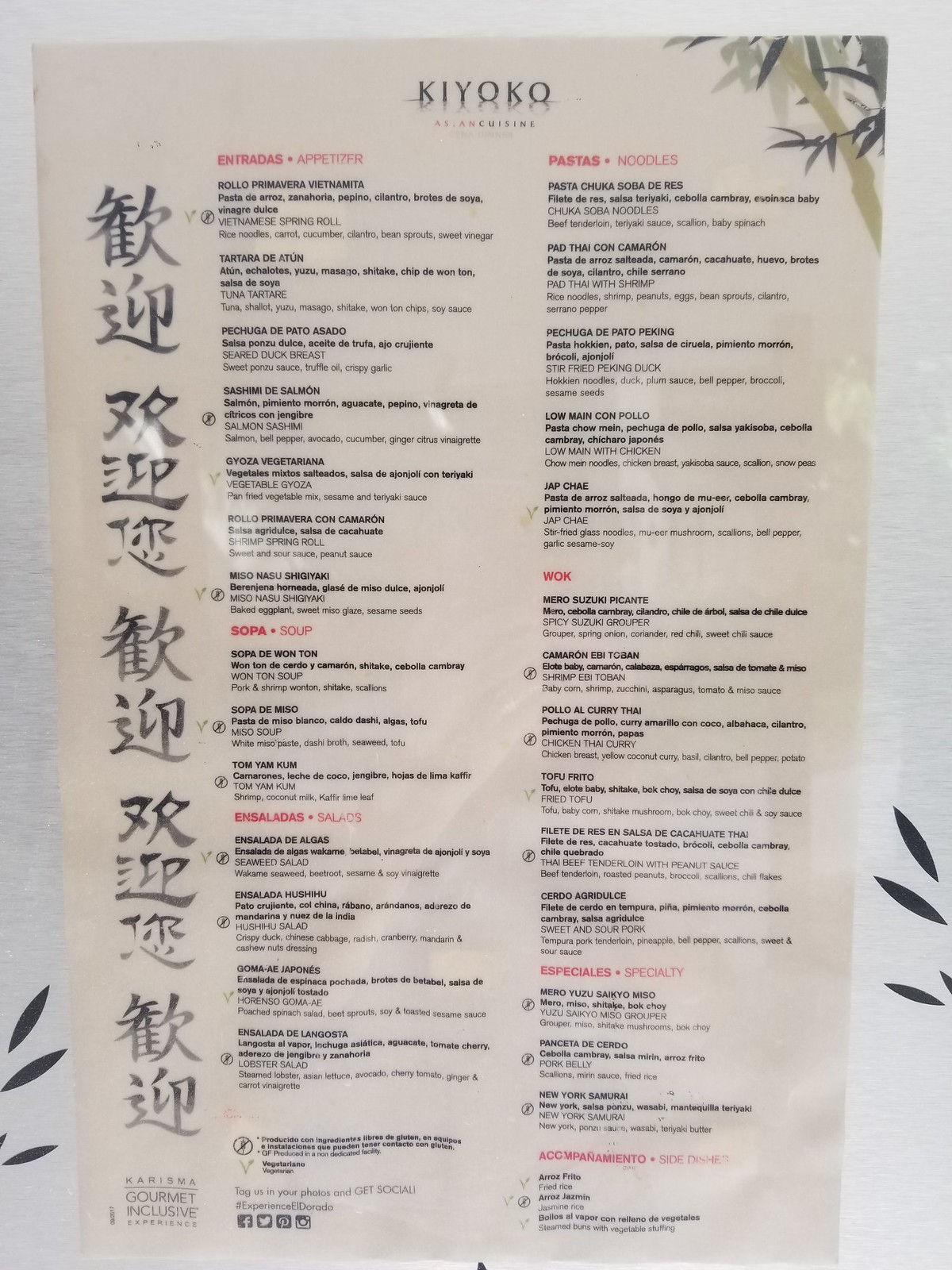The image depicts a restaurant menu printed on off-white paper, partially written in Japanese with some English terms. The menu appears to belong to a restaurant named "Kiyoko," as indicated by the prominent heading at the top. The text is in fine and small print, making it challenging to read the individual menu items clearly. The menu is organized into two columns, with dish types highlighted in red headers. In the left column, the headers are "Appetizer," "Soup," and "Salads." In the right column, the headers include "Noodles," "Wok," and "Specialty." The structured layout suggests a variety of traditional Japanese dishes and possibly some fusion offerings.